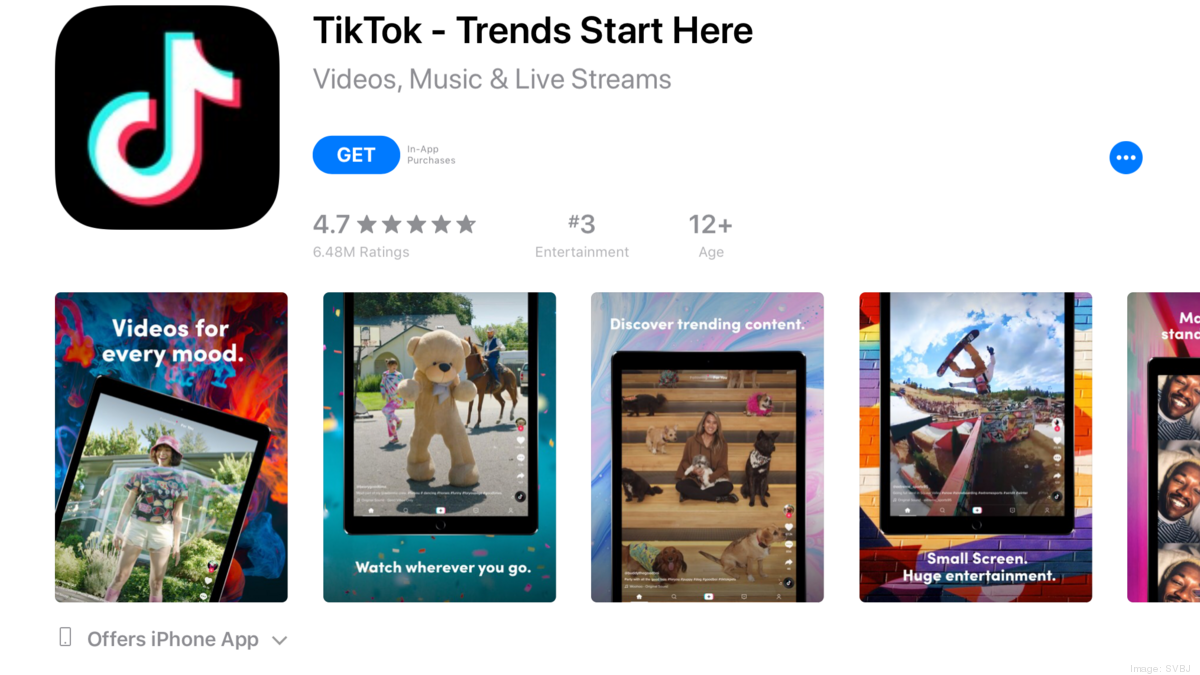A cropped screenshot from a digital device showcases a page from an application store featuring the social media app TikTok. In the upper left corner of the screenshot is TikTok’s distinctive icon—a sleek black square with a stylized music note in blue, white, and pink hues. Positioned prominently beneath the icon is a rating aggregate, displaying five grey stars paired with an impressive 4.7 score based on evaluations by approximately 6.48 million users. Directly below the rating are five individual images offering glimpses into the app's interface. Each image is a screenshot from within TikTok, depicting a range of video stills. Captions accompanying these images highlight TikTok's diverse features, including phrases such as "Videos for every mood" and "Discovering trending content," emphasizing the app's appeal and functionality.